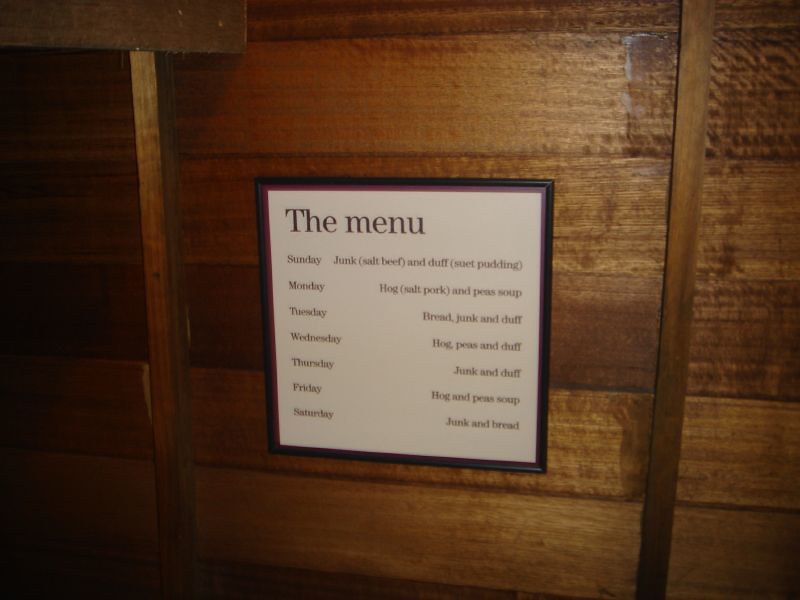This image captures a framed menu, meticulously hung on a wooden wall. The menu itself is printed on solid white paper with clear black lettering, encased in a sleek black frame. At the top, the title simply states "Menu." The days of the week, from Sunday through Saturday, are listed sequentially down the left side, with each corresponding day's meal extending to the right. 

For Sunday, the menu reads "junk, salt beef, and duff (suet pudding)." Monday offers "hog, salt pork, and pea soup." Tuesday's fare includes "bread, junk, and duff." Wednesday lists "hog, peas, and duff," while Thursday features "junk and duff." Friday repeats "hog and pea soup," and Saturday concludes with "junk and bread."

The menu is mounted against a backdrop of wooden planks that add rustic charm. The wall comprises both lighter and darker wood tones, primarily aligned horizontally. However, adding a unique architectural touch, two vertical planks intersect the horizontal ones, blending seamlessly in the same wood color tones. The contrast of the stark black and white menu against the varied wood textures creates a visually striking and historically nostalgic scene.